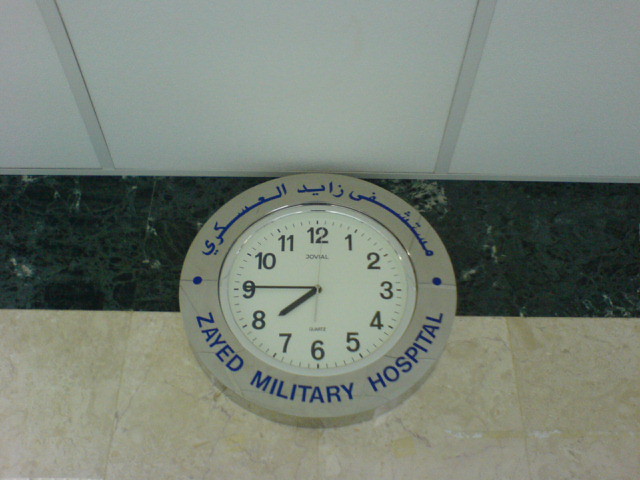This detailed photo captures a silver-bordered clock prominently positioned on a wall, near the ceiling. The wall itself is divided into two contrasting sections: an upper section of black granite and a lower section of white granite. The ceiling is lined with standard ceiling tiles. 

The clock face is encircled by a gray ring and features distinctive blue Arabic script curving around the top and blue English text at the bottom that reads "Zayed Military Hospital." The numbers, printed in black, outline the perimeter of the traditional clock face which also includes small dashes for minute markers. Below the '12,' in tiny letters, is the brand name "Jovial." The black hands of the clock indicate a time of 8:45. 

Additionally, there are notable design elements such as a blue dot positioned on either side of the clock face. The setting appears to be an Arabic-speaking environment, suggested by the script and the hospital designation. The accompanying floor consists of two different colored tile sections, featuring squares of beige, cream, off-white, with adjoining sections of black, dark green, and cream tiles, many scratched, further supporting the placement within a functional space like a hospital.